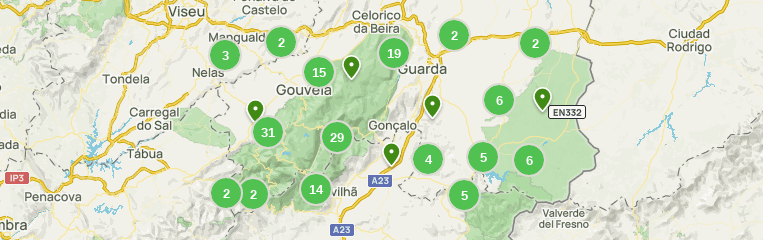The image depicts a rectangular map, likely a screenshot from Google Maps, featuring an area where the place names are predominantly in Portuguese, suggesting it could be Brazil. Topographic features are prominently displayed, including mountainous terrain, rivers, lakes, and various highways, depicted as squiggly yellow lines. In the central part of the map, there are several green circles with white numbers ranging from 2 to 31, with some numbers appearing multiple times. These circles are primarily concentrated in green-highlighted zones, which resemble national parks or natural reserves. Notable locations named on the map include Gouveia and Guarda. The overall layout shows a central oval-shaped green area with connecting diagonal and horizontal yellow roads, emphasizing the region's natural and infrastructural features.